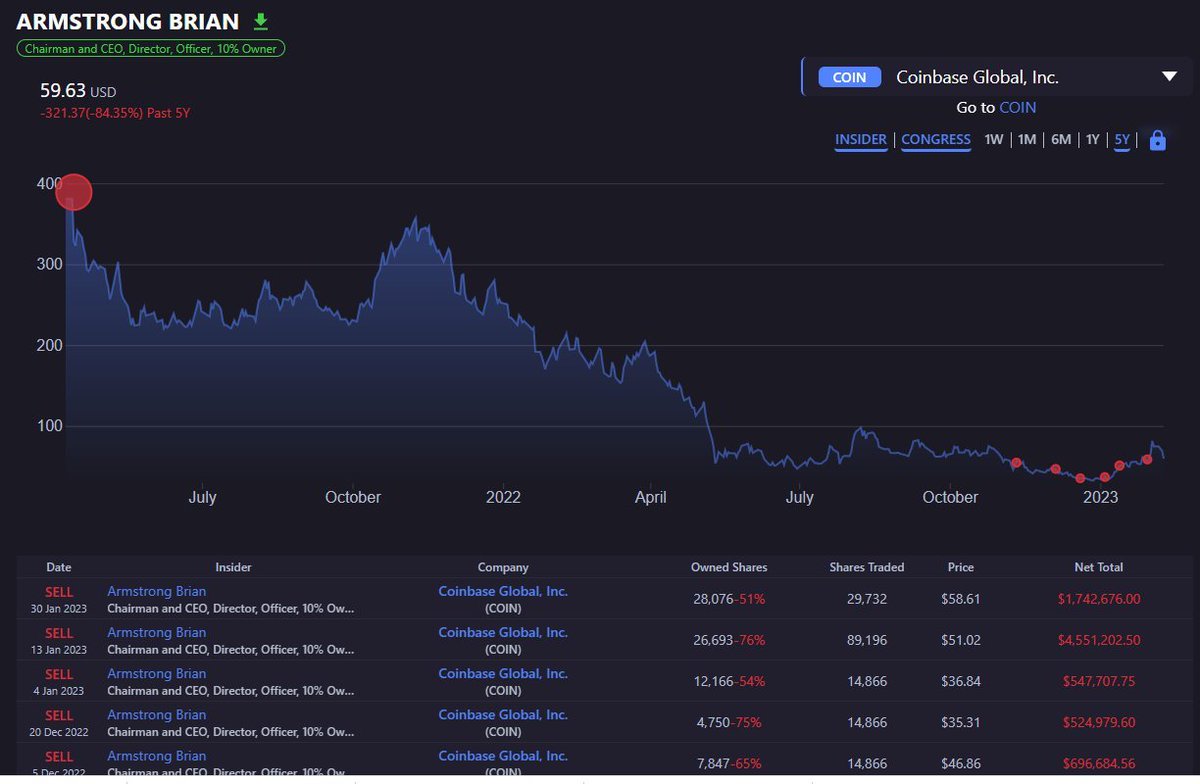The image depicts a screenshot from a financial website or application showing the stock performance of Coinbase Global Incorporated, listed under the stock name "COIN." The central feature of the page is a detailed line graph illustrating the stock's price trajectory over time, spanning from 2022 to 2023. At the beginning of this period, COIN's stock price was in the high range of $300-$400 per share. A large red circle in the top left corner highlights this high value.

However, the stock's value has significantly declined, with the current price noted as $59.63. Several dates in 2023 are also marked with red circles, likely denoting notable dips or critical events in the stock's performance.

At the bottom of the page, there is a list of individual transactions showing this user’s trading history. The list includes details such as dates of transactions, the company's name, the number of shares traded, the price per share, and the net total from each transaction. This detailed breakdown provides a comprehensive view of the user's interactions with the stock over the specified period.